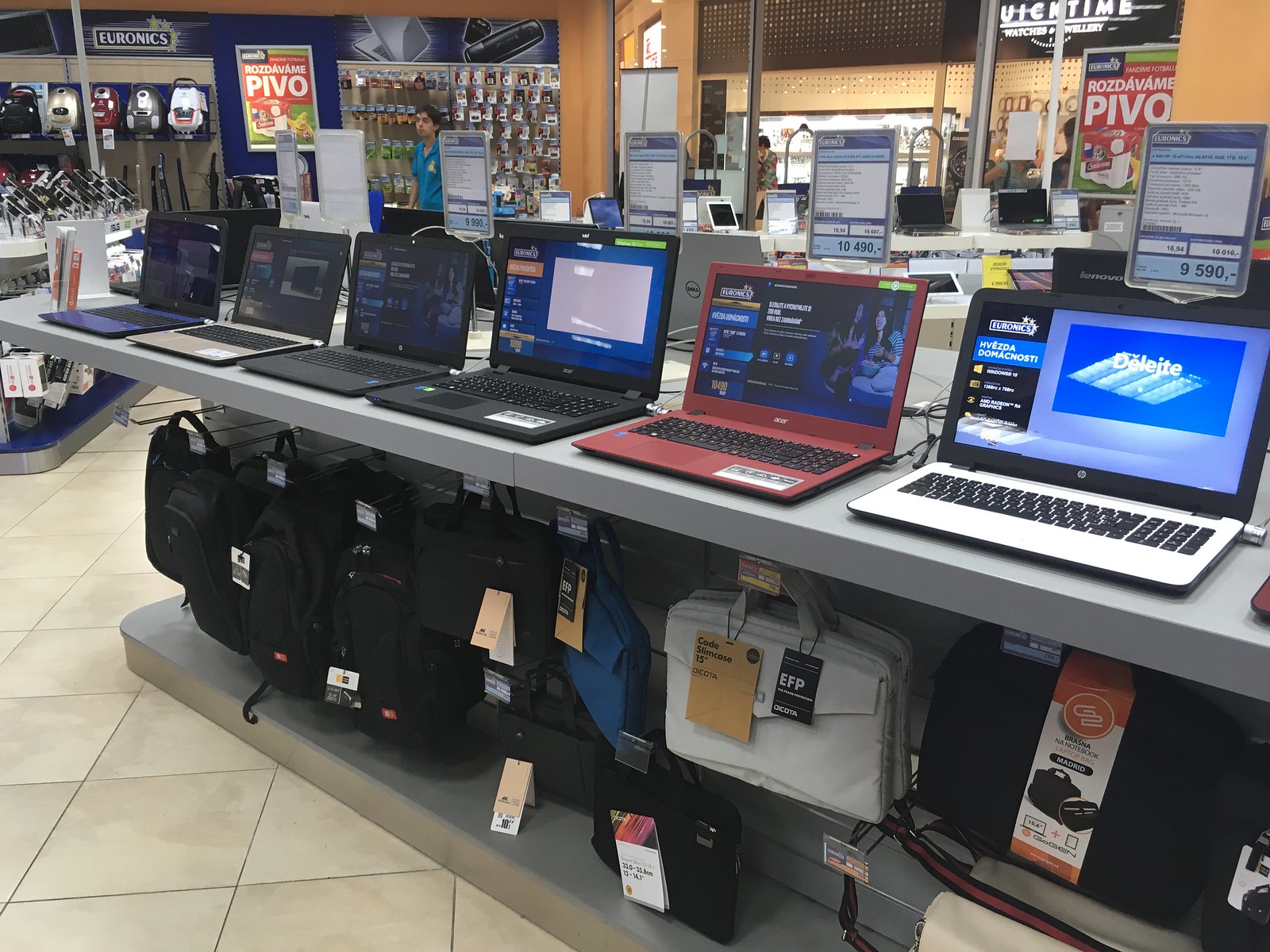The image is a color photograph taken inside the computer section of an electronic store, likely part of a larger mall given the visible glass window showcasing other stores in the background. The store has an 18 by 18 inch white ceramic tile floor and features gray display stands. On a prominent gray table in the foreground, there are several laptops of various sizes and colors, including black, silver, white, blue, and a striking red one. Each laptop is open with its screen turned on, and behind each one, there are informational tags with prices and specifications on metal stands.

Underneath the table, hooks hang from the wall holding various styles of laptop bags, including black backpacks, a white laptop bag, and a black crossover bag. Additional laptop cases in black, white, and blue are also displayed. Signs in the store read "Euronics" and "Pivo" in blue and white, with one sign featuring Cyrillic script that spells out "ROZHDAV". An area under the shelf displays even more zip-up laptop cases available for purchase. Toward the back, there is a salesperson or associate in a turquoise shirt, suggesting a customer service presence.